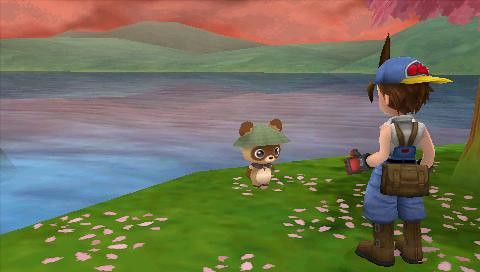This screenshot, likely from a video game reminiscent of an older Animal Crossing style, depicts a detailed and vibrant scene. The central figures include a boy, reminiscent of a Pokémon trainer, standing on green grass speckled with pink flower petals. The boy has short, spiky brown hair and wears a backwards baseball cap that's a mix of blue, red, and yellow, with a noticeable orange front. His outfit comprises a white t-shirt, blue overalls, and brown galoshes, along with a brown backpack. Interestingly, he sports an orange glove on one hand, giving a thumbs-up gesture.

Beside him stands an adorable teddy bear-like animal. This creature has a brown face with lighter tan-colored fur around its mouth and eyes, which feature a striking dark chocolate brown mask-like pattern. Its round ears taper into light gray at the base, and its belly and nose are beige-white, with the nose being distinctly black. The bear wears a cylindrical, straw-like green hat, adding a charming visual element.

In the background, a vibrant landscape unfolds with a tree adorned with pink and maroon leaves to the right. Beyond the characters, serene water bodies of light blue and dark grayish-blue hues stretch out, reflecting a dramatic sunset colored with orange, red, and purple hues. Rolling green mountains stand in the distance, completing the picturesque setting.